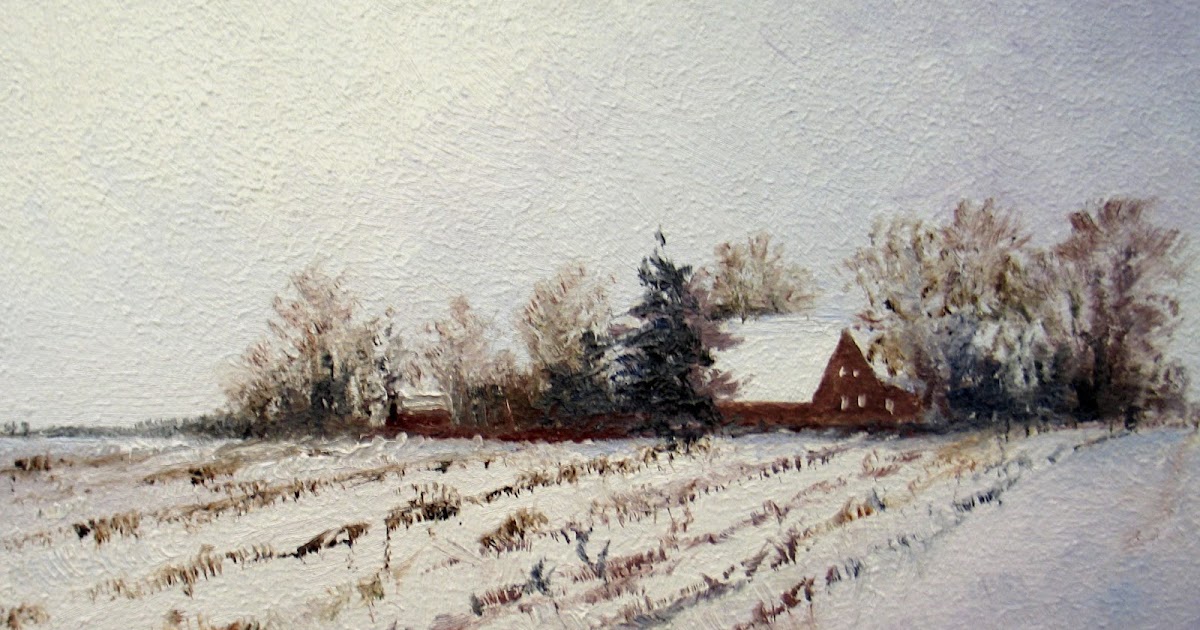The image is a created piece, likely a watercolor or pastel painting, depicting a winter farm landscape in a cold, snowy scene. In the center-right, there is a large, snow-covered farmhouse with a pointed roof, surrounded by various trees—a mix of deciduous trees with brown leaves and a lone evergreen pine. To the right of the farmhouse, there's a barn with a distinctive white roof, and a road running beside it. The foreground features rows of withered crops, likely corn, partially covered in snow, suggesting the recent onset of winter. On the left side, there's an open area that might be water, bordered by more trees with bare branches. The sky is a white-gray, adding to the chilly, wintry atmosphere. The textured background enhances the painted effect, emphasizing the unique and somewhat abstract artistic style.